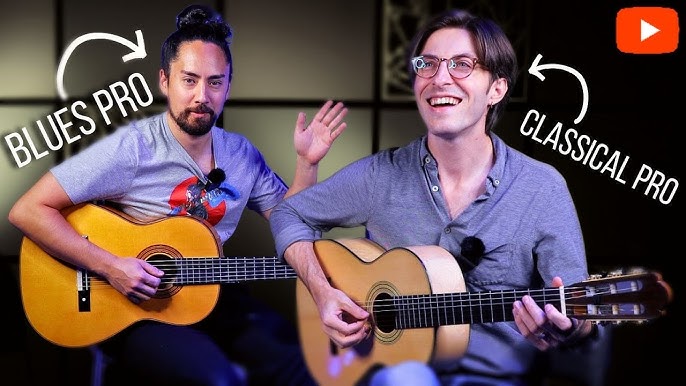This image appears to be a YouTube thumbnail for a video, featuring two men in what looks like a studio with soundproof tiles. Both men are sitting down with blonde wood acoustic guitars on their laps. The red YouTube logo with a white play arrow is prominently displayed at the top of the image.

On the left side of the picture, there is an Asian man with black hair pulled up in a bun, a black beard, and wearing a grey t-shirt with a red circular design that includes a person. He has a microphone clipped to his t-shirt and is waving with his right hand, while his left hand rests on his guitar. An arrow points to him, labeled ‘Blues Pro.’

On the right side, there is a Caucasian man with brown hair, glasses, and a longer hairstyle. He is smiling or laughing and looking off into the distance. He is wearing a grey button-up shirt with a microphone attached to the pocket, and blue jeans. Both of his hands are on his guitar, and he is seated in a black chair. An arrow points to him, labeled ‘Classical Pro.’

In the background, there is a white window that casts a shadowy effect, adding depth to the studio setting.